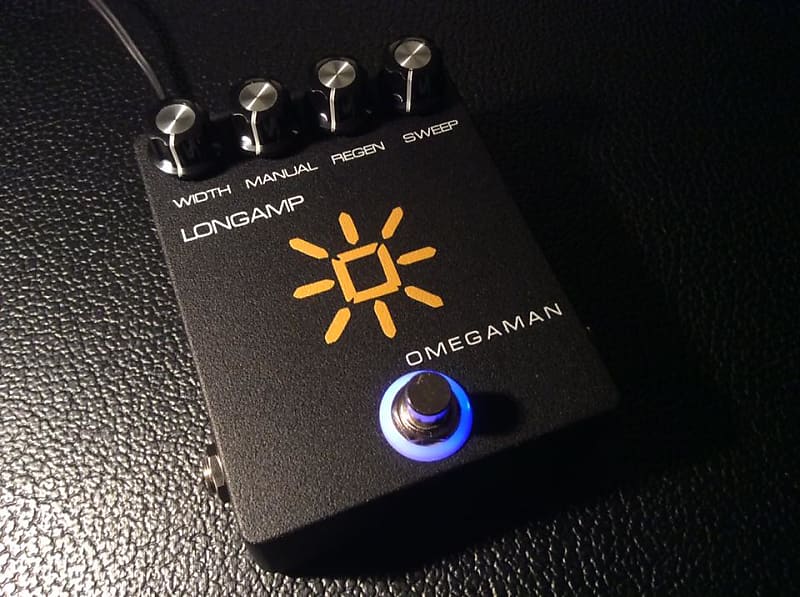The image depicts a black control device, likely a filter or pedal used for a musical instrument, such as a guitar. The device has a matte black finish, slightly textured, and is situated on a black, leather-like surface, possibly the top of a guitar case or amplifier. The device itself is slightly longer than it is wide and is positioned with a subtle tilt to the bottom left. 

At the top of the device are four black knobs, each featuring a silver top with a white stripe. Below these knobs are white labels: "Width," "Manual," "Regen," and "Sweep." Just beneath the labels for "Width" and "Manual," the brand name "Longamp" is inscribed in white lettering. 

In the center of the device, there is a distinctive yellow logo of a square-shaped sun with small orange spikes projecting from its corners and sides. Directly below this logo, the name "Omega Man" is prominently displayed in white text. Beneath the text, there is another black knob, encircled by a thin blue-lit ring, then a broader black area, and finally a light blue border encasing the knob.

A thin black cable extends from the top left corner of the device, indicating its connection to other equipment. The detailed design and the arrangement of controls suggest it is an interface meant for fine-tuning sound, most likely by a guitarist during a performance or recording session.